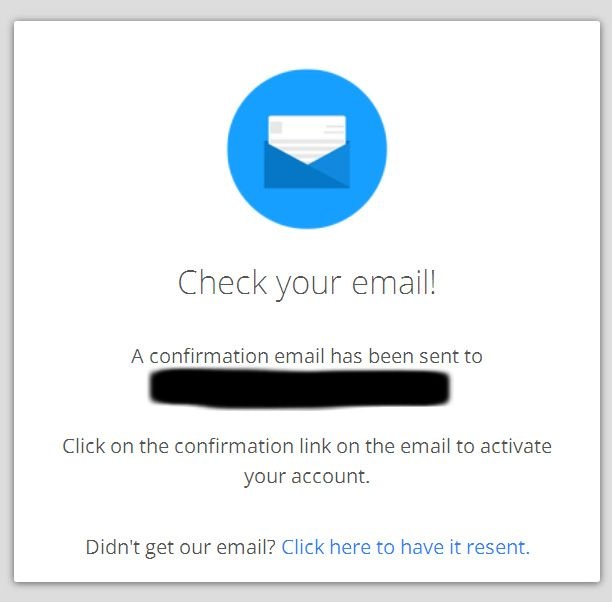The image displays a square-shaped pop-up notification centered within a medium grey background. The pop-up itself is white and outlined in dark grey. At the top center of the pop-up, there is a large blue circle containing a dark blue illustration of an envelope with a piece of paper emerging from it, featuring grey lines that suggest text.

Below this illustration, bold text reads "Check your email!" followed by a line space. The subsequent text states, "A confirmation email has been sent to [redacted email address]," where the email address is obscured with black paint. 

Another line space follows, and the next instruction reads, "Click on the confirmation link in the email to activate your account." There is yet another line space, leading to a smaller text that asks, "Didn't get our email? Click here to have it re-sent." The phrase "Click here to have it re-sent" is highlighted in blue, indicating it is a clickable link.

The origin, product, or website associated with this pop-up notification is not visible in the image.